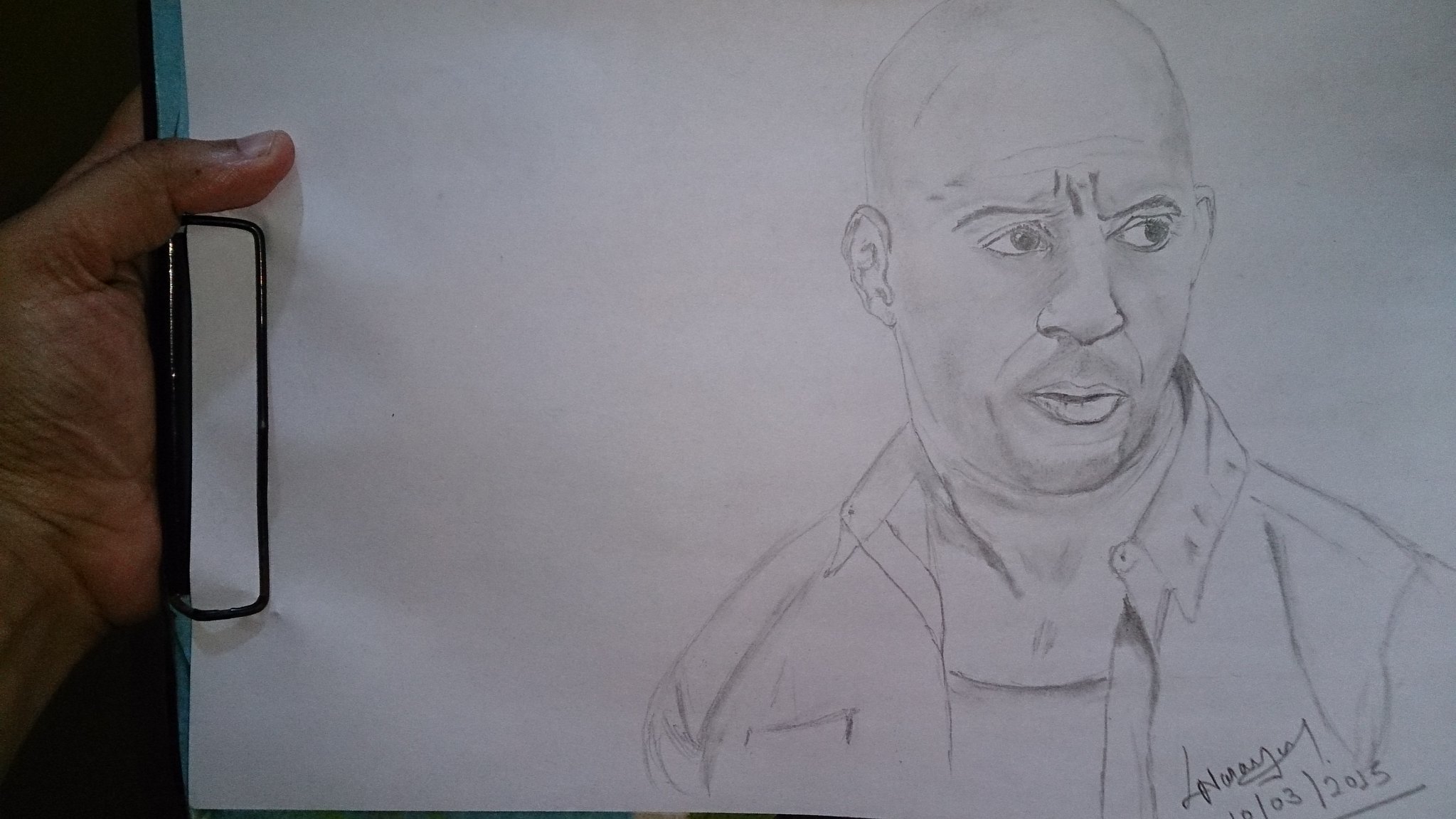A detailed pencil sketch of a bald-headed man is depicted on a piece of paper that is clipped onto a clipboard. A hand on the left side holds the clipboard steady. The man in the drawing is positioned on the right side of the paper, gazing to his right with a concerned expression. Delicate shading highlights his light wrinkles around the mouth and forehead, adding depth and realism to the sketch. He wears a collared shirt, casually unbuttoned, with a tank top underneath. The artist's signature and the date are neatly inscribed in the bottom right-hand corner of the paper. The drawing exhibits fine pencil work, illustrating both the textures of the man's clothing and the contours of his face and neck.